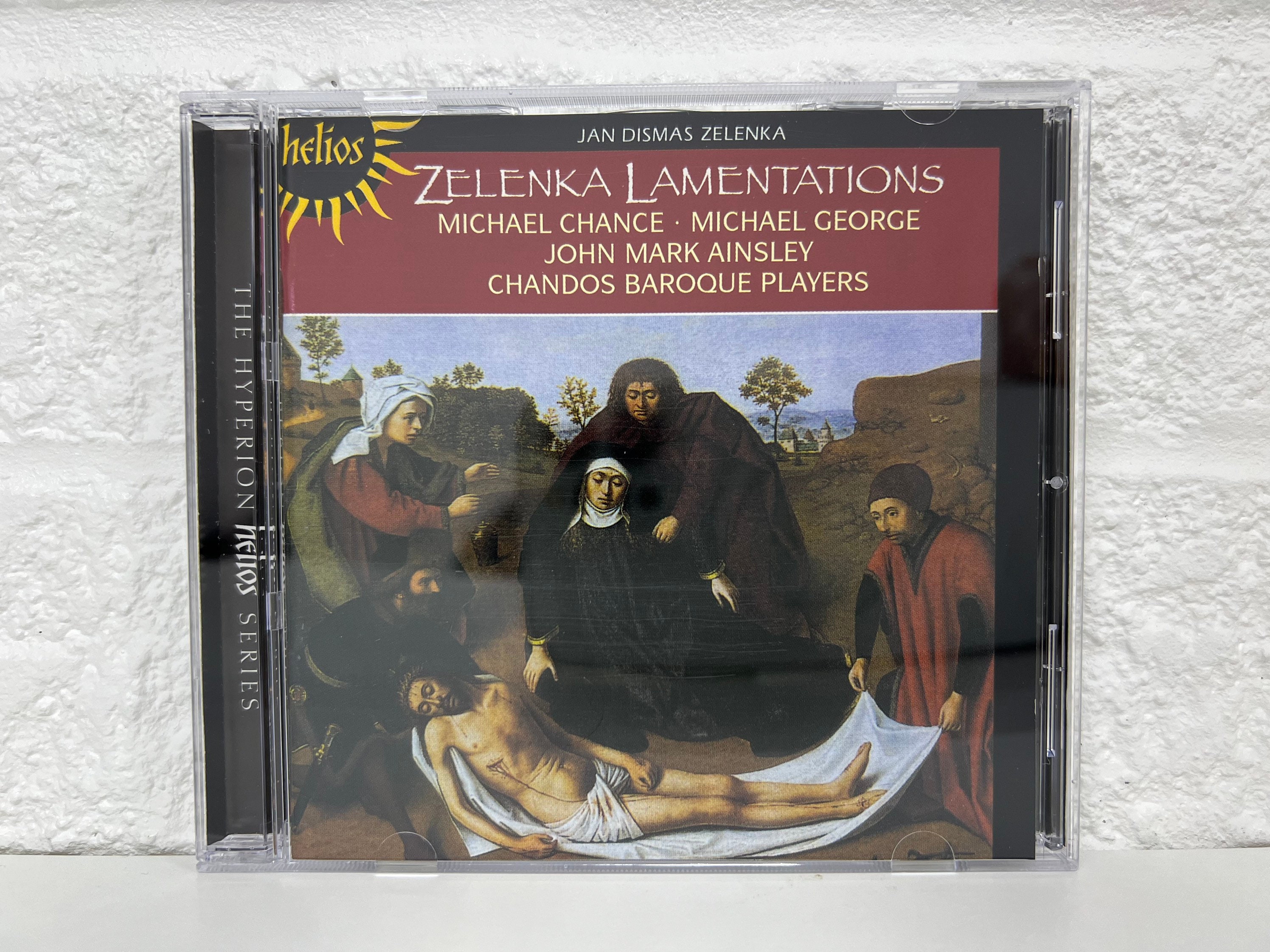This detailed color photograph showcases a music CD in a clear plastic jewel case, set against a white brick wall. The CD features the album "Lamentations" by John Dismas Zelenka with performances by Michael Chance, Michael George, John Mark Ainsley, and the Chandos Baroque Players. The cover art forms part of the Hyperion Helios series, prominently displayed with the Helios logo—a yellow sun with flames on a black background.

The CD cover itself resembles a Renaissance painting of Jesus being taken down from the cross and laid out on a white cloth. Jesus, depicted either suffering or deceased with closed eyes and a noticeable wound dripping from his left chest, is draped in a white cloth around his groin and another one beneath him. To his right, a man assists with the cloth, while at the center, a woman dressed in a black habit stands distressed, being comforted by a man behind her. To the left side of the image, another man holds the cloth, accompanied by a bearded man in black and a woman in a white headscarf and red-sleeved dress. The painting’s background features small trees, a brown landscape, and a blue sky, adding to the somber yet serene atmosphere of the scene.